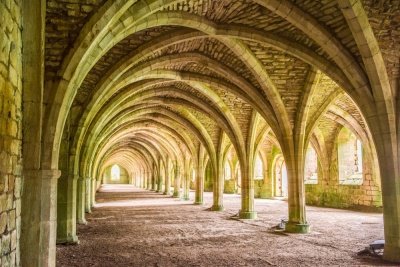This image depicts a medieval-looking setting, possibly computer-generated, resembling an underground or courtyard area of a castle. The scene features a series of stone pillars and arches, which create a vaulted, cylindrical space reminiscent of catacombs or a vast corridor. The stone pillars, made from brownish stone with green moss-like accents, support the structure, while the ceiling is composed of curved stone or brick patterns that intersect perpendicularly, forming a complex web of arches. Light filters through some window openings on the right and at the back, illuminating the area with a yellow-green tint. The floor appears to be composed of gray dirt, enhancing the aged and authentic medieval ambiance.